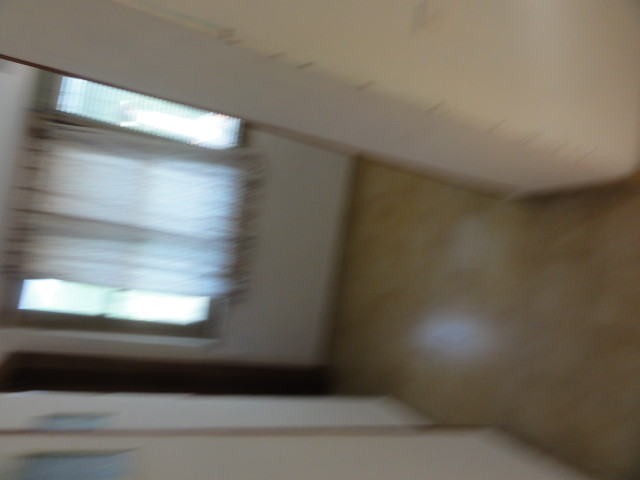The image is a blurry, motion-captured photograph of a room's interior, possibly a bedroom or a space that once was or will be a bedroom. The room appears to be located in a basement, suggested by the unusual structural angle of the ceiling and a low-hanging, wide overhead section that indicates a walking area or hallway above. The walls are brown with a marbled appearance, while the front-facing wall of the room features two white walls with brown borders, framing a central window. 

The window, which looks out to a daylight setting with potentially visible trees, is covered with disheveled Venetian blinds that are closed but unevenly gathered in the middle. The flooring is peculiar, with wide stairs that descend but abruptly end at the wall under the window, adding to the room's ambiguous purpose. Given its layout and features, it might serve as a spa or jacuzzi room.